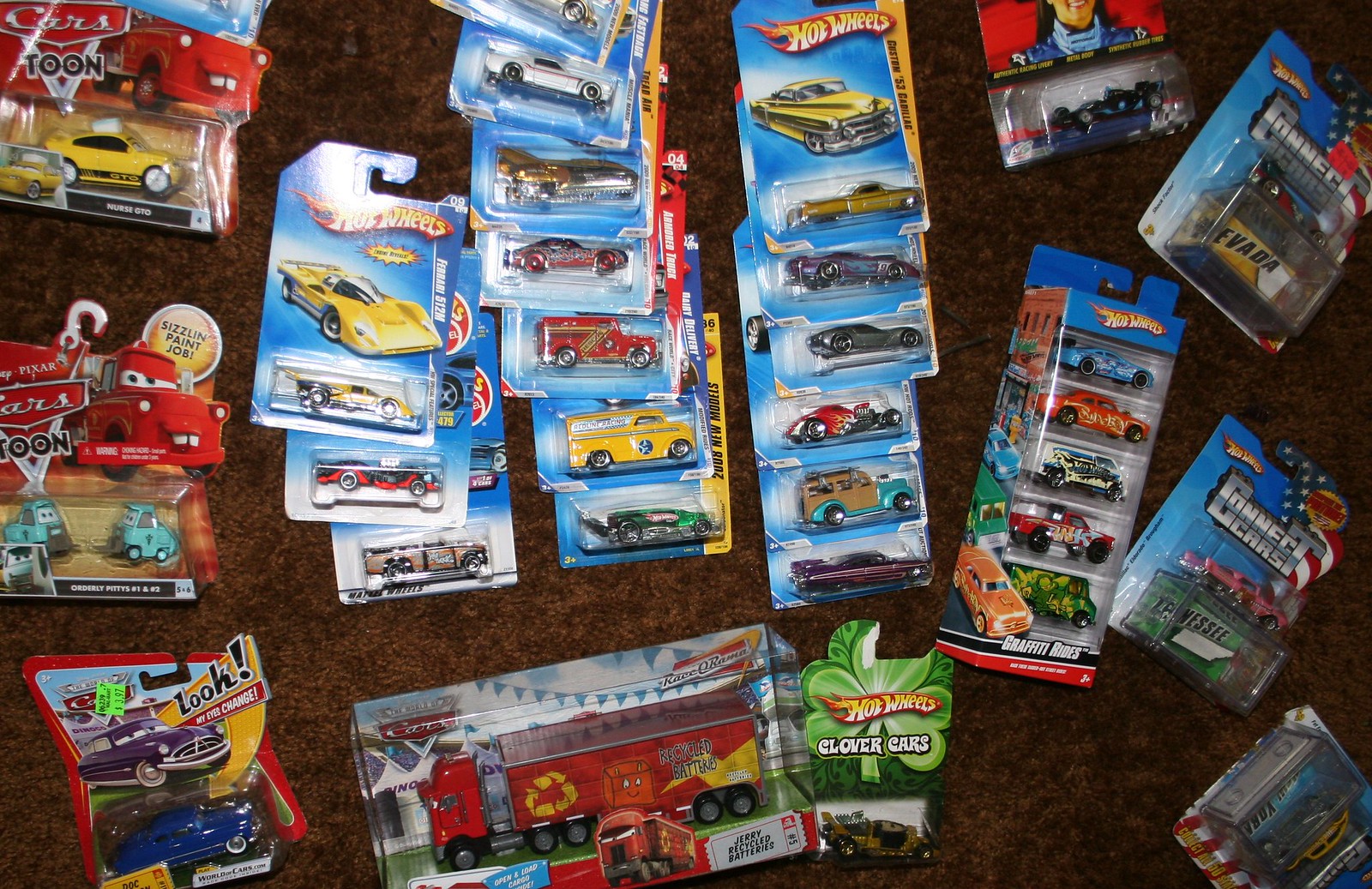This image showcases a diverse collection of Hot Wheels cars meticulously arranged and still in their clear plastic packaging, attached to cardboard backings. The cars are laid out flat against a rust-colored shag carpet, suggesting a collector's careful display. On the left side, there are three packages branded with notable model names. In the center, three columns exhibit varying numbers of Hot Wheels cars: the leftmost column has three, the middle column boasts seven, and the right column contains six packages. To the right, four additional packages are labeled as Connect cars. Adjacent to these is a multi-pack of Hot Wheels, along with two more packages at the bottom. The cars range from iconic Ferraris and a classic panel truck to a fire truck and a blue tow truck character from Pixar’s animated film “Cars.” The bright colors of the collection stand out vividly, including a yellow sports car and a green clover-themed car, adding to the visual splendor of this meticulous collector’s display.